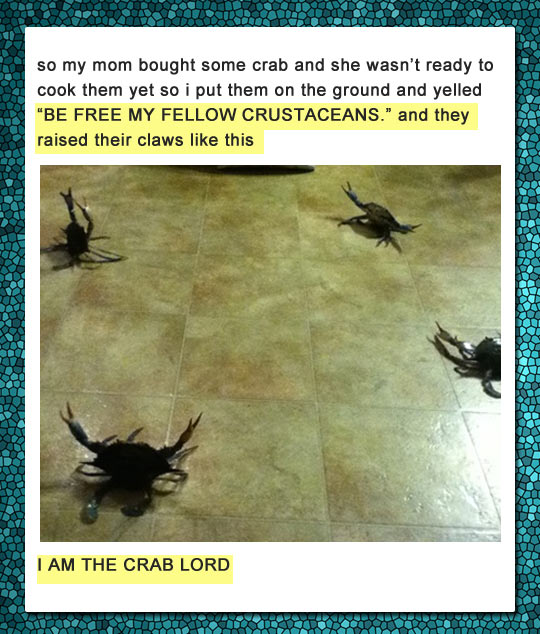In this indoor colored photograph, probably taken in a kitchen, four black crabs are seen crawling on a brown, tiled floor. Each tile is about one square foot, arranged in a five by five pattern. The photograph is framed by a decorative blue border resembling tiny stones and further bordered by a plain white rectangle. Above the image, in black text, it reads, "So my mom bought some crab and she wasn't ready to cook them yet so I put them on the ground and yelled, 'Be free, my fellow crustaceans!' And they raised their claws like this," with the phrase "Be free, my fellow crustaceans! And they raised their claws like this" highlighted in yellow. Below the image, the caption continues in all capital letters, "I AM THE CRAB LORD." The crabs, three of which have their claws raised, are positioned with one in each corner and one slightly above the bottom right corner, giving a humorous and lively effect to the scene.